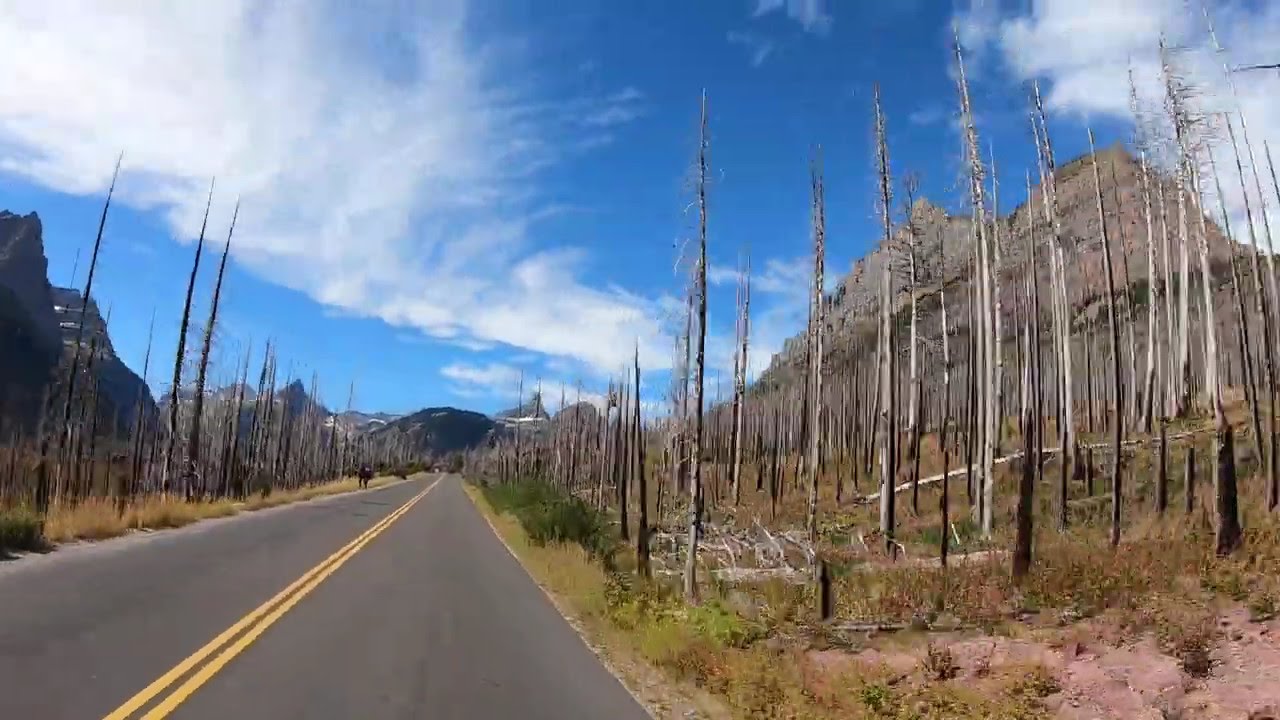A photo taken from inside a car captures a long, two-lane paved road with a central yellow double line stretching far into the distance, flanked by a forest of barren, burnt trees. The landscape hints at a recent fire with the bases of the trees blackened and devoid of branches and foliage. Green grasses and shrubs skirt the reddish-brown dirt lining the road. Towering on both sides, the rugged granite mountains showcase dramatic peaks and tan slopes streaked with brown. The sky overhead is a vibrant blue, dotted with scattered white clouds that drift across the frame. In the far distance, the road leads towards a series of mountains on the horizon. Two people can be seen ahead, capturing photos of the majestic scenery. Among the distant details, a tiny, indistinct figure—possibly an animal—stands on the side of the road, adding a mysterious touch to this panoramic scene.